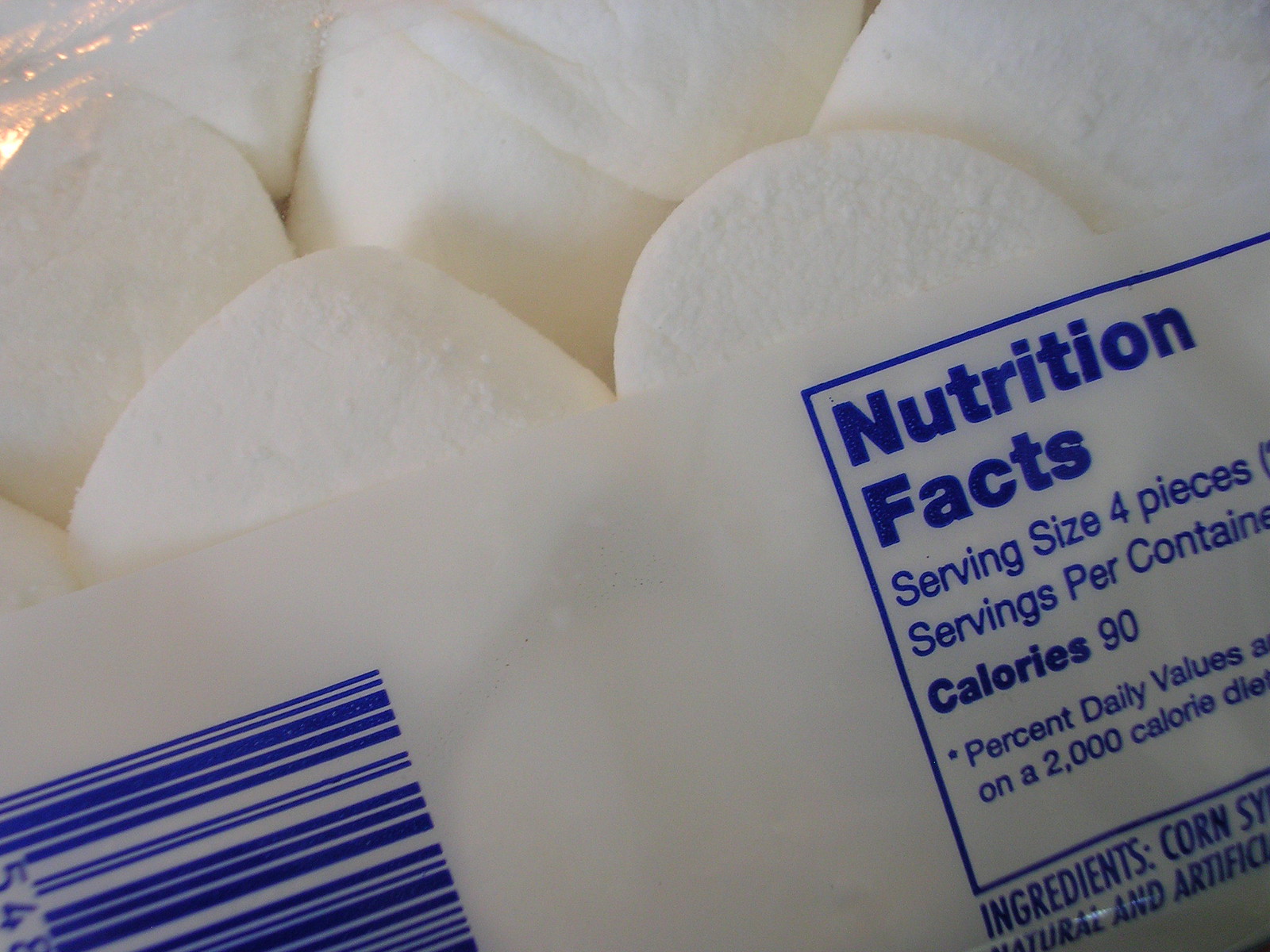This is a very close-up photograph of a bag of marshmallows. The upper half of the image is dominated by large, fluffy white marshmallows, arranged on a slant. Below the marshmallows, there is white plastic packaging that spans the bottom half of the image. On the lower left-hand side, there is a partially visible blue barcode. To the right, there is a blue-framed area containing nutritional information. The text within this area, written in blue, reads: "Nutrition Facts," "Serving size: four pieces," "Servings per container," "Calories: 90," and "Percent daily values are based on a 2,000-calorie diet." Due to the angle and proximity of the shot, some portions of text are cut off, including the ingredients list, where only parts of words like "corn syrup," "natural," and "artificial" are visible.